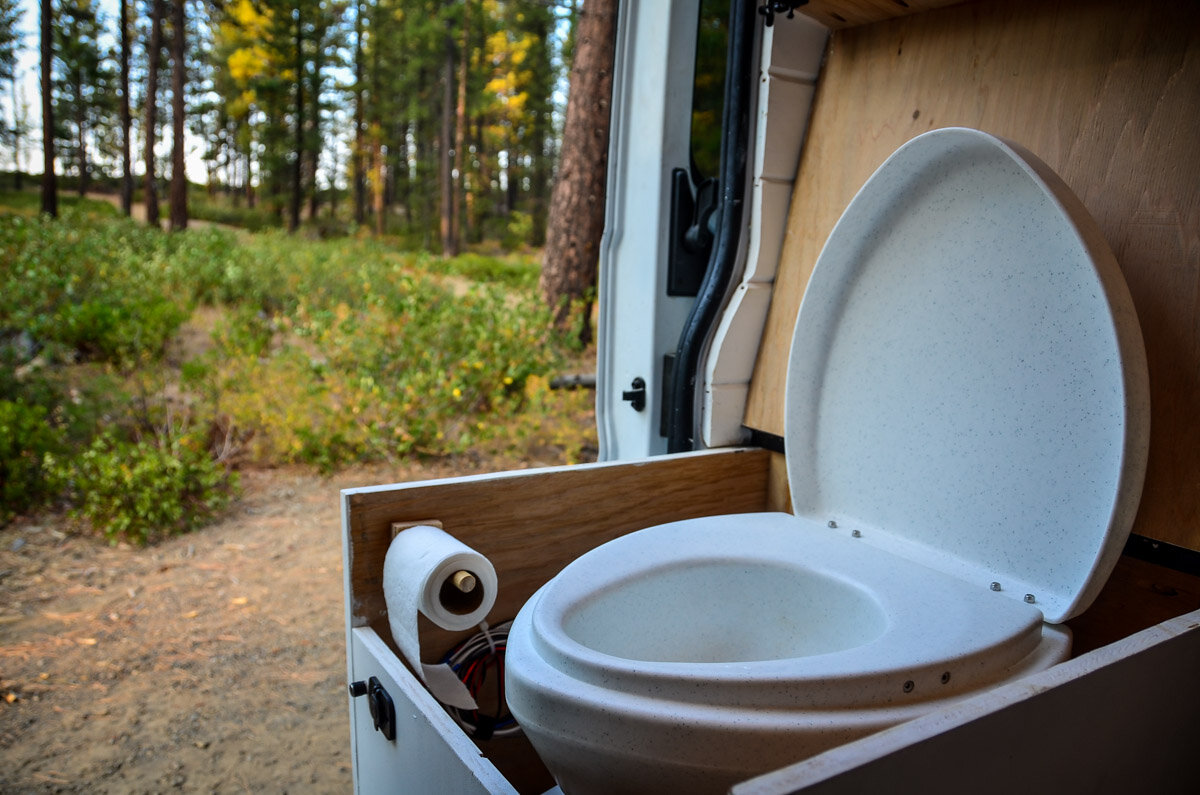This photo captures a unique blend of indoor and outdoor environments, featuring a portable toilet set within a van that's parked in a wooded area. The van door is open, creating a seamless transition between the interior and the exterior. The toilet, which is the focal point of the image, is housed in a wooden box with a white lid that's currently open. Attached to the wooden box is a roll of white toilet paper. The box has a white door with a black latch on the front. Behind the toilet, there's a wood plank and some white tiles, enhancing its makeshift yet functional design. To the right of the setup, you see part of the van's metal structure with white framing. The left side of the image reveals the natural surroundings with tall trees, patches of grass, dirt, and glimpses of the sky peeking through the canopy. The overall scene is slightly blurry but clearly depicts a sunny day, emphasizing the peculiar indoor-outdoor bathroom arrangement.